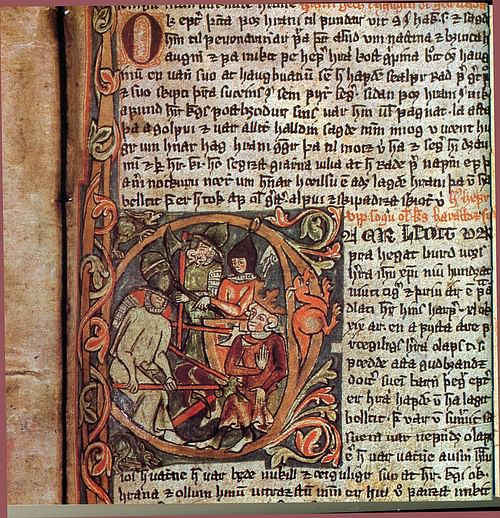The image depicts a very old, vintage page, likely from a medieval manuscript. The intricate black writing at the very top of the page is detailed and ornate, with highlighted text in both red and orange hues. An enlarged, ornate 'O' in red with an orange background is prominently located on the top left side. The left side of the page also features a detailed square illustration depicting what appears to be medieval soldiers or royalty amidst intricate vines. The central narrative portrays a group of medieval figures, adorned in various colored outfits, including red, orange, and green. Some figures are armed with weapons like axes and spears, all wearing helmets, suggesting a possible battle scene. The language of the text appears ancient and unidentifiable, adding to the historical ambiance of the image. The clarity of the image is high, with the detailed, aged craftsmanship visible under bright, natural lighting.